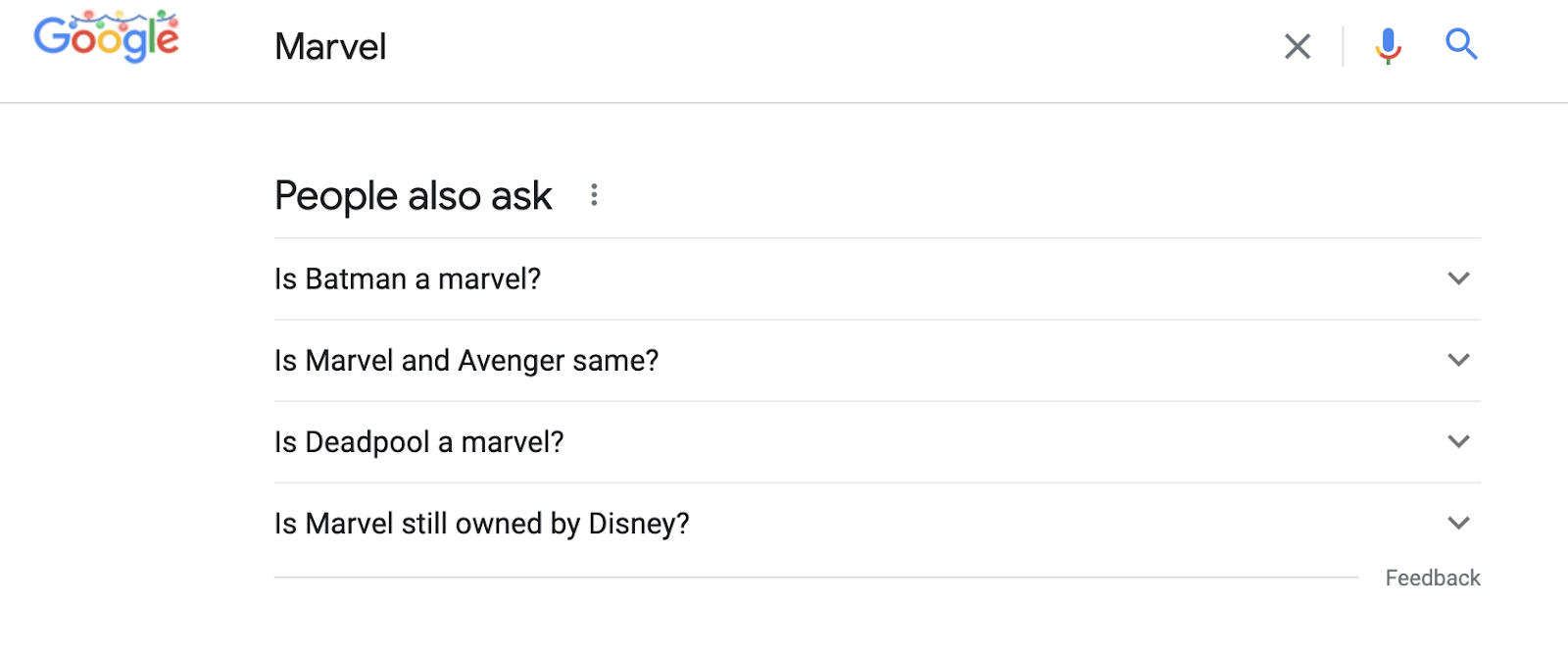The image is a screen capture of a Google search page. At the top of the image, the iconic multicolored Google logo is displayed, with each letter in blue, red, gold, blue, green, and red respectively. Above the logo, a string of Christmas lights is depicted, consisting of a blue string adorned with blue, red, green, and yellow circular bulbs.

Below the Google logo, there is a white search box containing the word "Marvel" in black text. To the right of the text, there is a gray "X" icon for clearing the search term, followed by a colorful microphone icon in shades of blue, gold, red, and green for voice search. A blue magnifying glass icon, symbolizing the search function, is also visible nearby.

Beneath the search box, there's a thin gray line, separating the search field from the rest of the content. The results section begins with the heading "People also ask" in black text, accompanied by three vertical gray dots.

The search suggestions are individually separated by thin gray lines and feature pull-down arrows next to them. The suggestions listed are:
1. "Is Batman in Marvel?"
2. "Is Marvel and Avengers same?"
3. "Is Deadpool a Marvel?"
4. "Is Marvel still owned by Disney?"

At the bottom, there is a "Feedback" link in gray text, with the "F" capitalized.

The overall quality of the image is excellent, with sharp, bold fonts that are easy to read and visually accessible, with no pixelation or blurring. The contrast between the black text and white background enhances readability, making it user-friendly, especially for individuals with low vision.